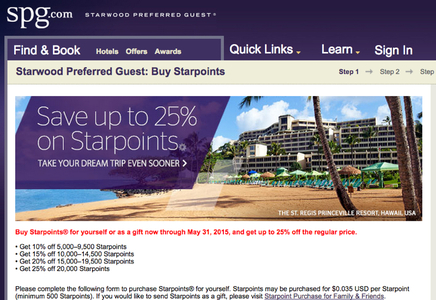The image is a colored advertisement for SPG.com (Starwood Preferred Guest), showcasing their online platform for booking hotel stays, offers, and award points. The homepage provides an option to sign in, indicating it is a generic page accessible to anyone before logging in. A prominent banner, overlapping an image of an expansive beach resort, captures attention. The resort is grand, with approximately 10 levels, each featuring windows that offer spectacular ocean views. The beach scene includes typical lounge chairs and umbrellas set against a picturesque ocean backdrop.

The banner headline encourages visitors to "Take your dream trip even sooner," emphasizing the opportunity to save up to 25% on Star Points. Customers have the option to purchase Star Points for personal use or as a gift, with a special offer valid through May 31, 2015. This promotional message is highlighted in bold red text, underscoring the urgency and appeal of this limited-time deal. Additional website features mentioned include tools to find and book hotels, explore special offers, and buy Star Points directly from the site.